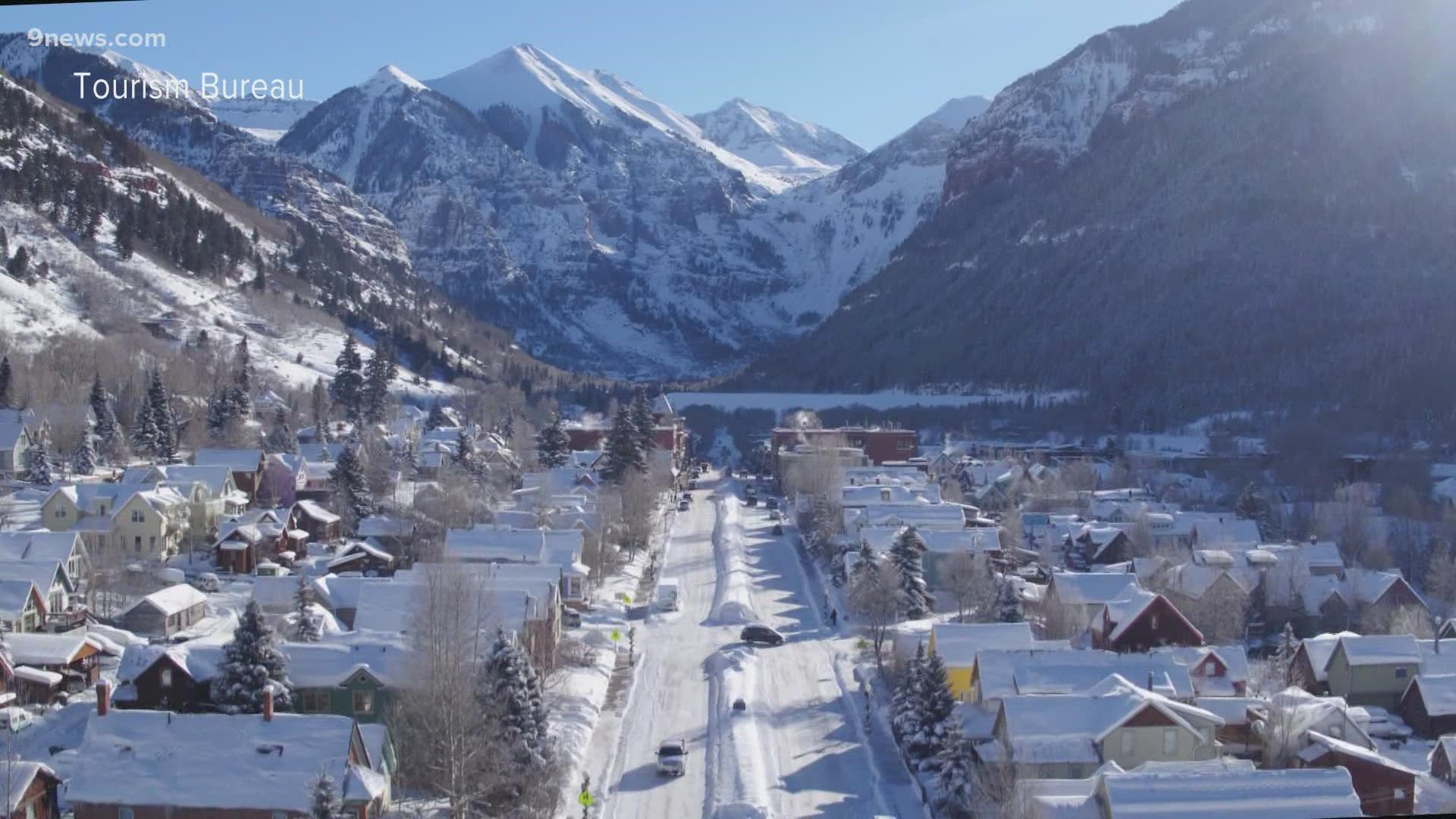This overhead high-angle shot captures a bright, sunny winter day in a cozy, inviting village nestled in a snow-covered valley between towering, snow-capped mountains. The village, featuring traditional, colorful houses, stretches up to the feet of these large, rocky peaks. A four-lane main street, heavily laden with snow despite evident plowing, runs from the bottom of the image through the heart of the village towards the mountains. The scene also features snow-laden pine trees and barren trees, contrasting with the vibrantly-colored houses. Vehicles traverse the snow-covered streets, adding to the bustling yet tranquil atmosphere. The upper corners of the image bear the watermark "9news.com Tourist Bureau," further framing this picturesque winter scene under a clear blue sky.